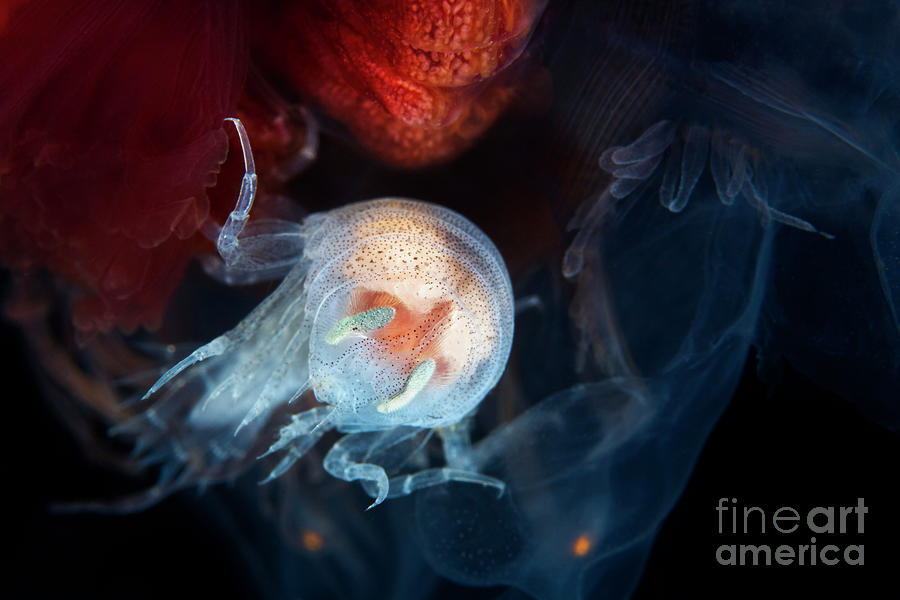In this vividly colored, animated underwater scene, a glowing, semi-translucent jellyfish-like creature takes center stage, resembling a ghostly apparition. The main body of the creature is bluish on the inside, surrounded by a translucent white and adorned with tiny black speckles. Its trailing, tentacle-like appendages, some of which are lifted like legs, extend to the bottom left of the image, with greenish antennae or feelers visible near its head. The jellyfish emanates a warm reddish-orange glow at the top, contrasting with its cooler blue hues. This scene is set against a predominantly black background, punctuated by semi-transparent, bluish, smoky shapes. Additionally, there are patches of red light at the top middle and top left, providing a dynamic and mysterious ambiance. The image is artistically rendered, with the lower right corner marked by the inscription "Fine Art America" in gray letters.